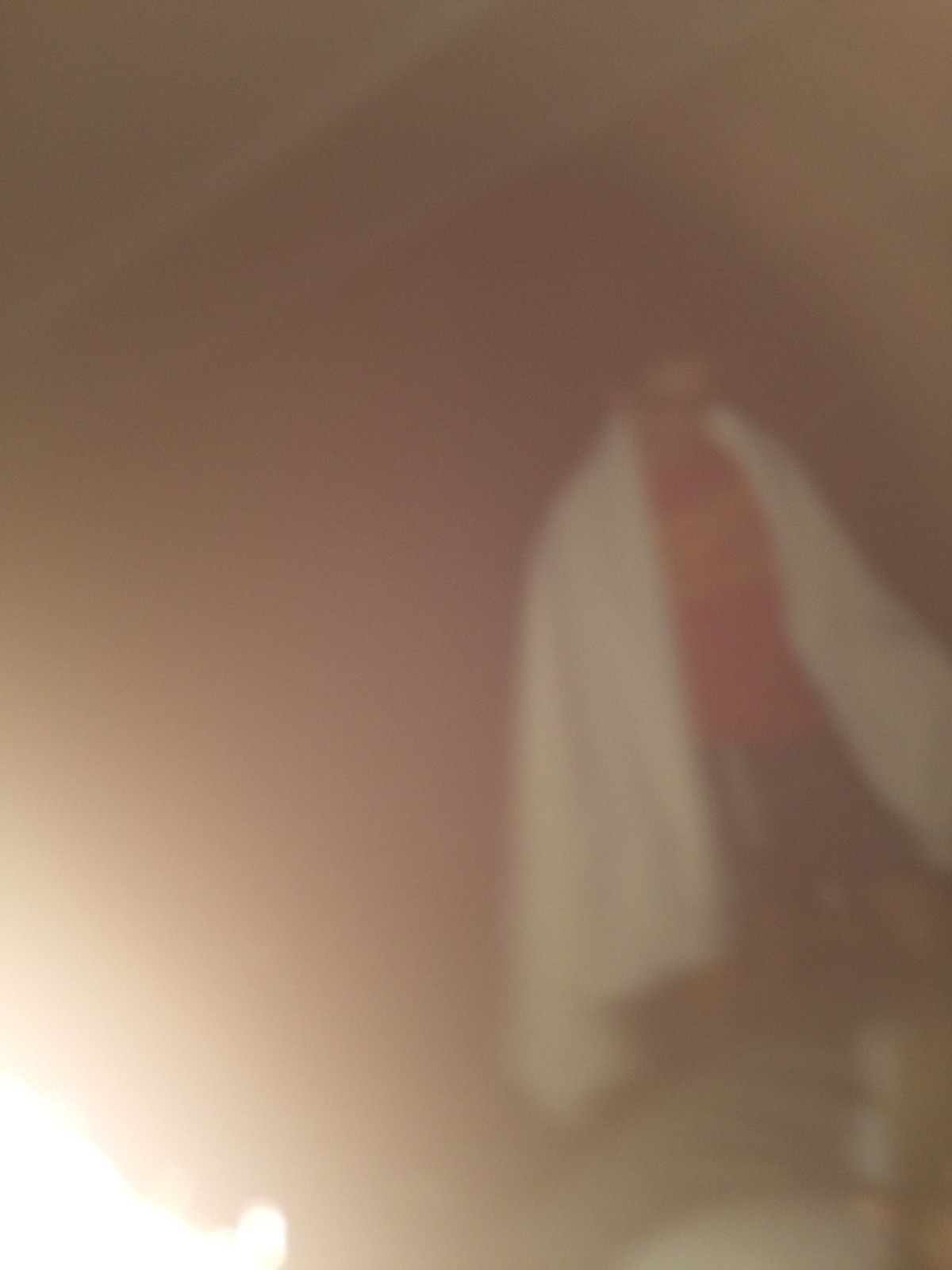This out-of-focus photograph features a man wearing glasses, standing slightly off-center in what appears to be an attic room with A-shaped ceiling beams. He is dressed in a red t-shirt that might have yellow writing or a logo on it, and has a long white blanket or towel draped over his shoulders. The image is heavily affected by a bright light source in the bottom left corner, creating a significant glow that washes out much of the picture, leaving the rest of the scene darker in comparison. The overall blurriness and high contrast due to the light make it difficult to discern further details.